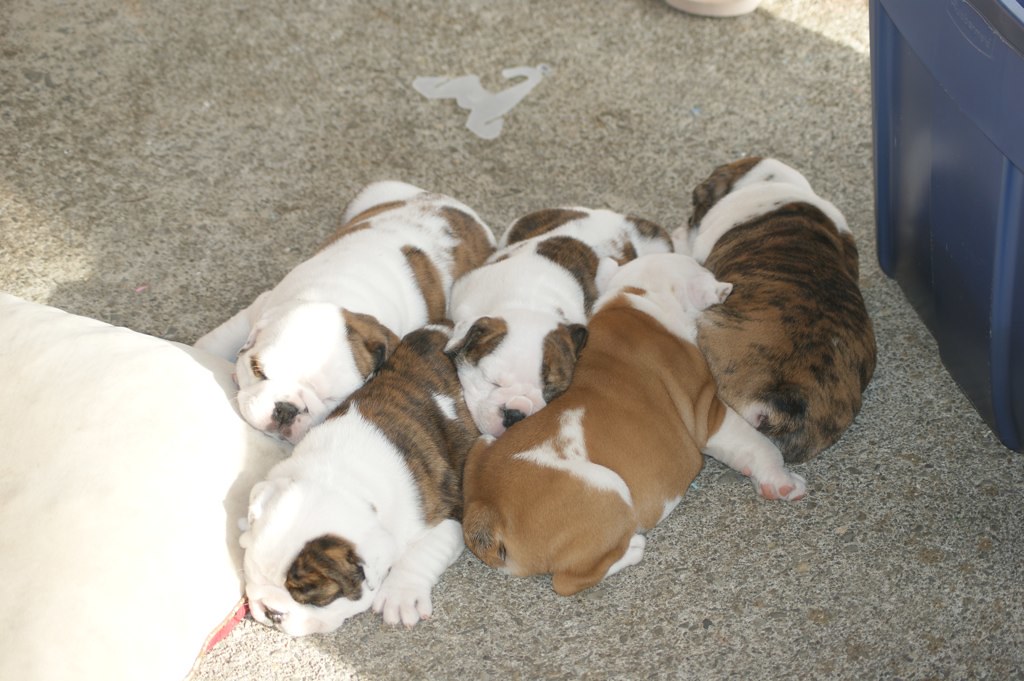This photograph captures a heartwarming scene of five sleeping English Bulldog puppies nestled together on a light gray carpet. The puppies display a delightful mix of white and brown colors with some showcasing darker brown stripes and brindle patterns. Three of the chubby, squishy-faced puppies are adorably facing the camera, allowing a clear view of their black noses and the endearing folds in their faces, particularly around their left eyes. The other two puppies have their backs to the camera, exposing their small tails. To the lower left, a white doggie bed peeks into the frame, while a dark blue storage container sits to the right. The entire scene is bathed in a soft light, possibly from a nearby window, highlighting the peaceful slumber of these charming bulldog puppies.